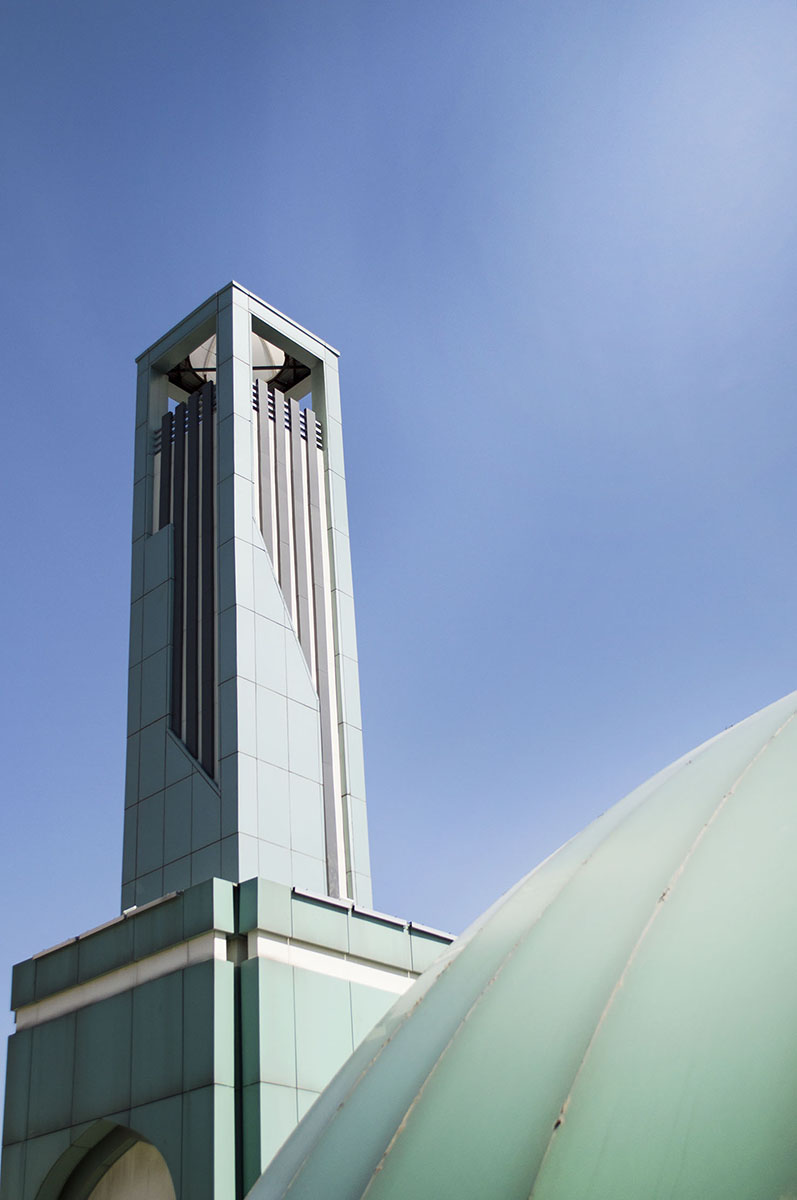The image depicts a photograph of a distinctive architectural structure set against a clear, cloudless, light blue sky. The focal point of the image is a bell tower perched atop a larger building. The building exhibits a predominantly light green hue with a hint of blue, and is constructed mainly from vertical rectangular bars. The bell tower itself is characterized by large wood-like slats and sits on a slightly thinner base. A prominent white dome caps the tower, which features black rails running across openings on all sides, giving it a distinctive appearance. 

To the lower right of the frame, there is a circular part of the building that extends upward slightly below the center right edge and down past the bottom center, hinting at the presence of a large green dome that might serve as an entrance or another functional area of the structure. Near the top edge of the square base, an indented white bar adds architectural interest. Overall, the photograph conveys a sense of place, likely captured during a visit, with its clear and detailed focus on the building’s unique design elements.